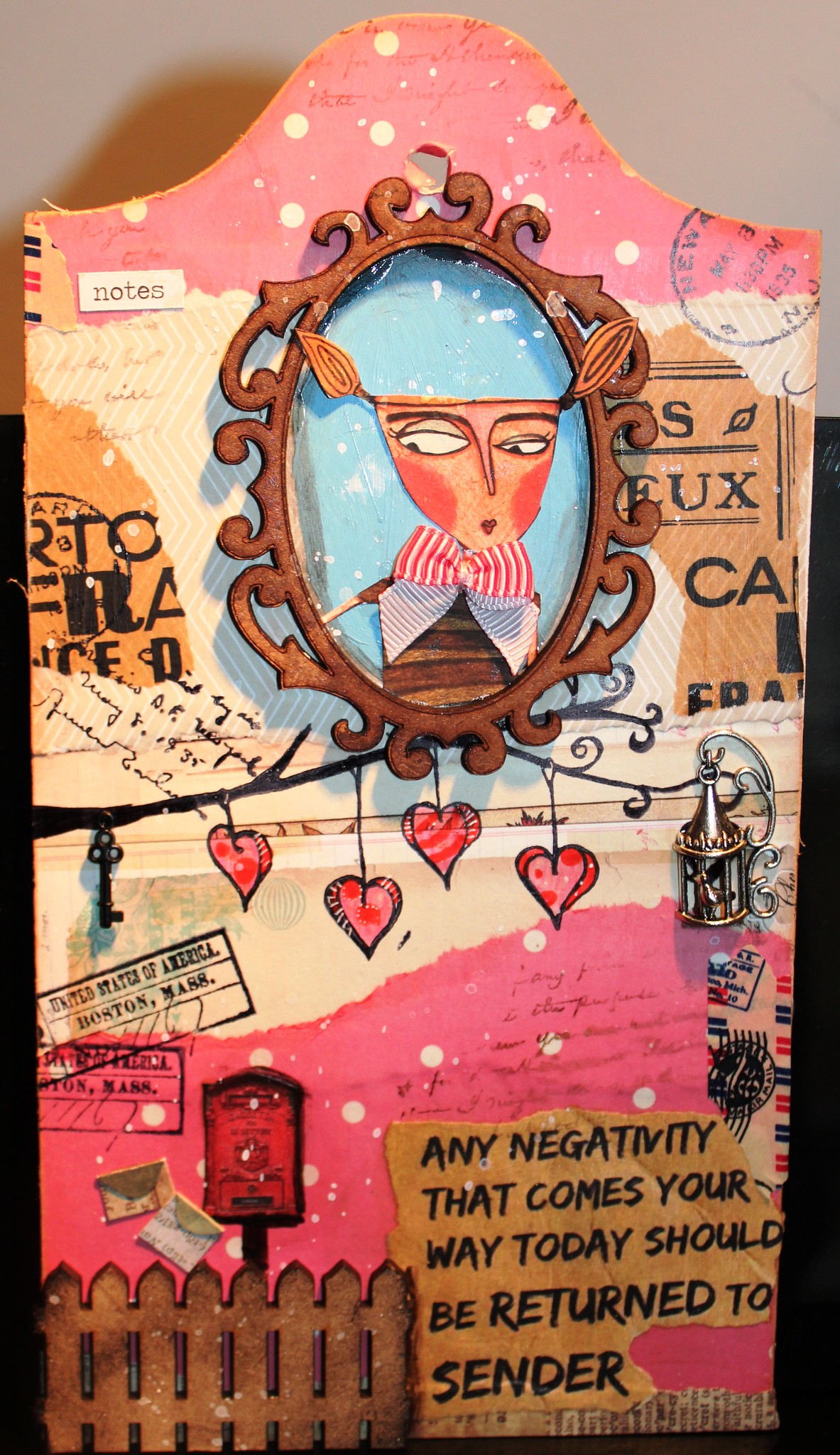This eclectic collage artwork, shaped as a tall, rectangular piece with a scalloped wave at the top, is designed as a humorous greeting card. The image is replete with intricate details and various media elements. The background transitions from a tan color at the top one-third to a stark black below, while the artwork itself is set against shades of pink and white. 

Centrally, an ornate filigree picture frame with a scrolling wooden design houses an unusual figure—a hybrid of a deer and a person—donning a red, blue, and white striped tie and a bow tie. The figure's eyes gaze sideways, emerging from a mirror-like portal. Above them, squiggly pigtails suggest a playful touch. 

To the right side of the frame, delicate features such as a tree branch with small red hearts and a hanging key add to the whimsical nature. The tree branch contrasts against a brown picket fence in the lower left corner, accompanied by a red mailbox displaying some letters. Scattered above are various words and a postmark in the upper right corner that reads "Newark, N-E-W-A, May 8th, 1935, New Jersey."

The bottom of the artwork includes textual elements: "United States of America, Boston, Mass" and the phrase, "Any negativity that comes your way today should be returned to sender," printed in black on a brown background in the lower right corner. This multifunctional collage combines humor, nostalgia, and artistic flair in a singular, cohesive display.